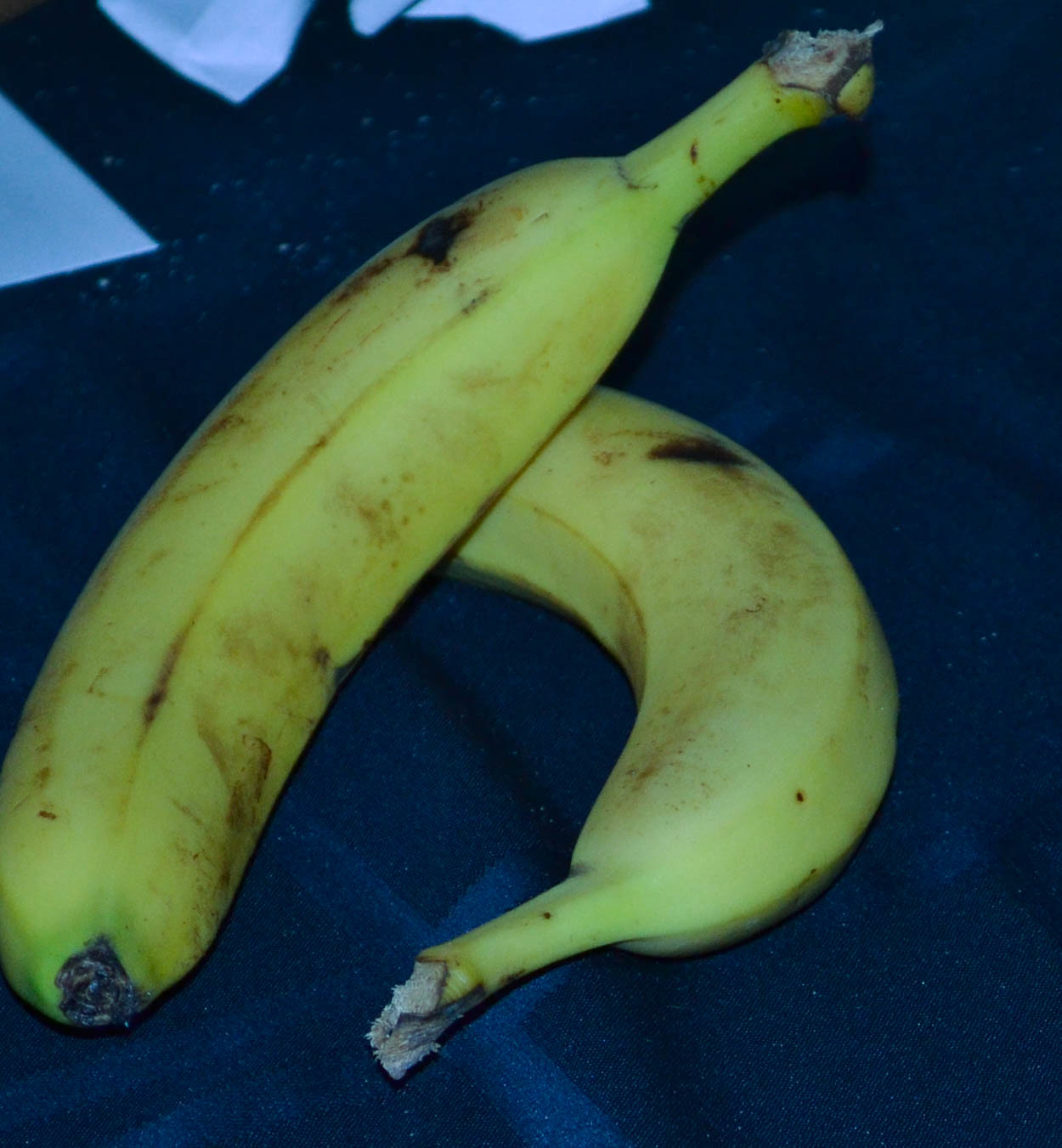On a mysterious, navy blue background with hints of lighter blue in the top left corner, two bananas take center stage. The bottom banana, visibly detached from its bunch, starts from the middle of the image slightly to the left and gracefully curves to the right. It displays a mixture of ripeness, with brown spots dotting its yellow skin and hinting at overripe areas. Above it lies the second banana, positioned in the top left corner and curving upwards in a sleek, comma shape towards the right. This banana, too, has brown spots scattered across its surface, indicating the early stages of overripeness. The end of its stem slightly protrudes, resting gently on the bottom banana, creating an intriguing, layered composition.